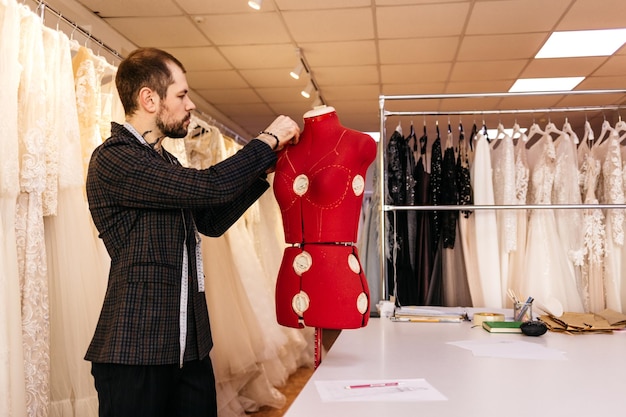The image captures a meticulous tailor or fashion designer, distinguished by his dark, checkered-pattern suit jacket, black trousers, and white or grey shirt. He has brown hair, a matching mustache, a brown beard, and neck tattoos, exuding a confident persona. The scene unfolds in a bustling fashion workshop where the designer is intensely focused on a red dress form, draping fabric and adding detailed stitches that outline the chest and waist areas. His hand rests thoughtfully on the shoulder of the mannequin, which showcases a high-neck outfit with a belt and circular silver or white elements. The workspace features a large white work table filled with various objects and is surrounded by racks of clothing, including red and black dresses. Behind him, a whole row of lacy white dresses, presumably wedding gowns, emphasizes his expertise in bridal fashion. This highly detailed setting underscores the designer's role in crafting or fitting wedding dresses.